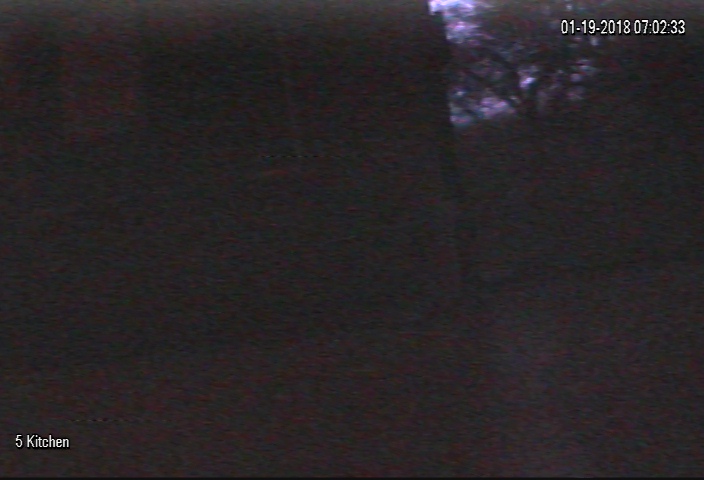This image depicts a very dark and blurry photograph, taken outside at night. Dominating the left-hand side of the photo is a structure, possibly the corner of a house or building, which appears black and indistinct. Within this dark area, there is a faint outline that might be a window. Surrounding the structure, particularly towards the right, the photograph shows a hazy sky with subtle shades of blue, gray, pink, and hints of purple, possibly indicating the presence of sunrise or sunset hues. In front of this sky, the branches and leaves of a few trees are visible, though they remain blurry and undefined. The bottom part of the photo is a slightly lighter shade of black, hinting at the presence of a ground or road. In the upper right corner, there is a time and date stamp reading "01-19-2018 07:02:33." Additionally, the bottom left corner features a small white text indicating "5 Kitchen," which might be related to a security camera designation. The overall image is shrouded in darkness, making the identifiable details scarce and indistinct.